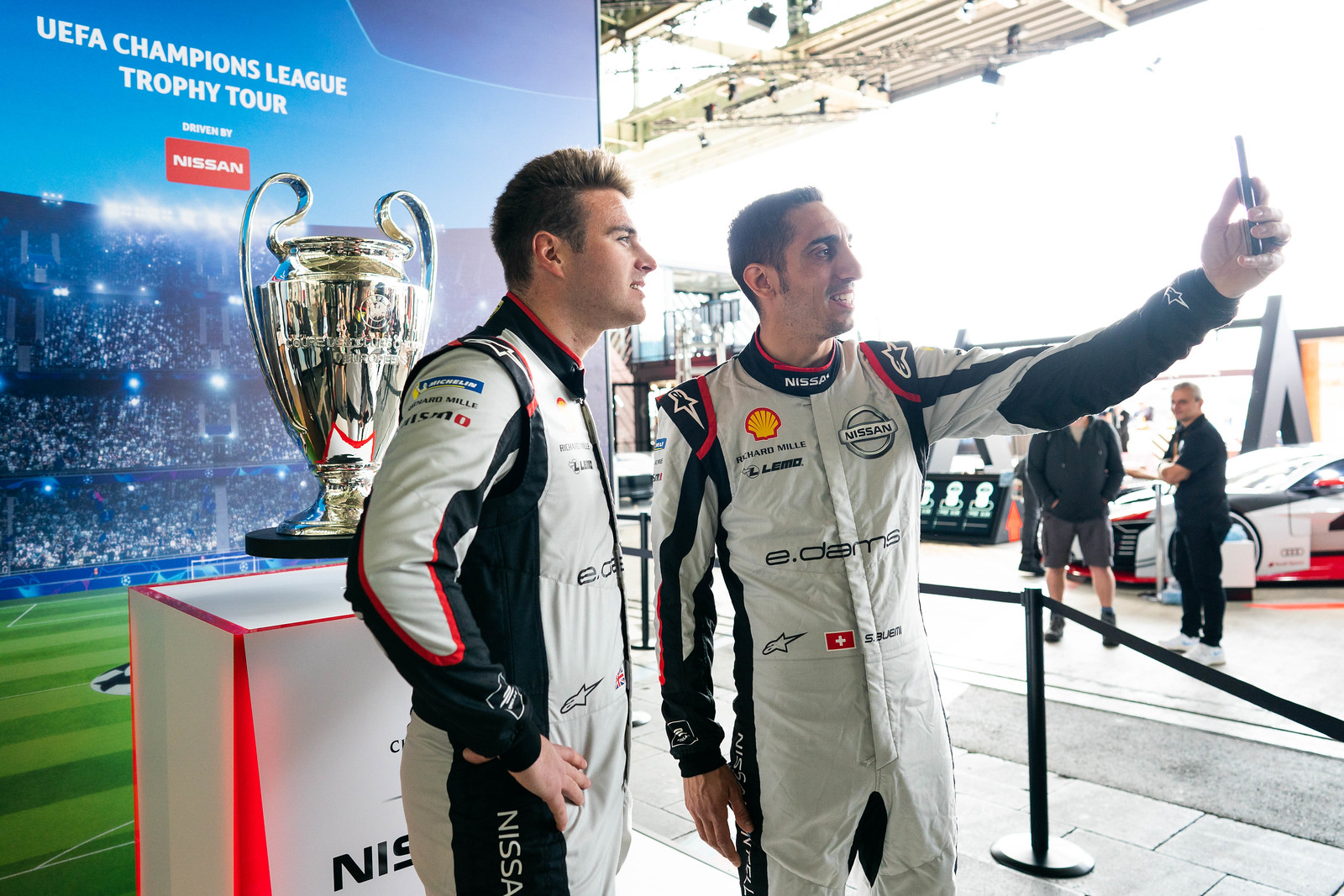The photograph captures two young men, likely in their 20s, who are standing in front of the UEFA Champions League Trophy Tour backdrop. Both are dressed in racing suits - predominantly light gray with black sides and arms, accented by red collars. Their uniforms proudly display multiple sponsor logos, including prominent placements for Nissan and Shell Oil Company, indicating their athletic status, possibly as race car drivers.

The man on the right extends his left arm to take a selfie, while the man on the left stands with his hands on his hips, looking at the camera. Behind them stands the centerpiece of the event: a large, shining silver trophy, seemingly hovering above its stand. The backdrop features a sign that reads "UEFA Champions League Trophy Tour" with the Nissan logo in bright red. Adjacent to them, the scene extends into a larger venue, possibly a white hangar, with a race car visible and a few onlookers in the distance. A barrier marked by poles and a rope separates the two selfie-takers from the background onlookers. The entire setting is bathed in ample light, suggesting either a vast window or an exterior setup, adding a glary brightness to the photograph.